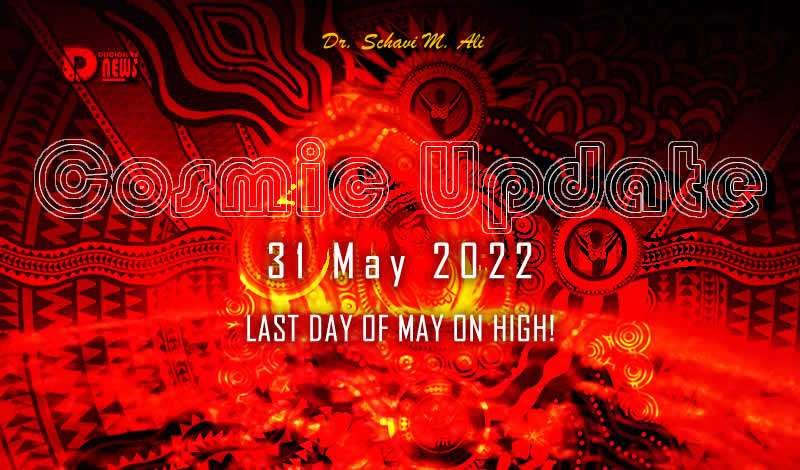This advertisement for Dr. Schavi M. Ali prominently features his name in elegant yellow cursive lettering at the top of the poster. Below, the text "Cosmic Update" stands out in large, psychedelic white letters with intricate outlines. This is followed by the date, "31 May 2022," and the emphatic phrase, "Last Day of May on High!" all centrally justified. The background is a dynamic blend of fiery red and black, with hints of yellow, featuring various cosmic shapes and symbols—circles, triangles, and complex patterns that evoke a glowing, almost planetary design. Despite their intricate forms, these shapes are difficult to distinguish as they blend seamlessly into the fiery backdrop, lending an almost mystical feel to the advertisement. In the upper left corner, there's a red "D News" logo with a black outline and an underline beneath "News," adding a further layer of detail to this complex and eye-catching design.